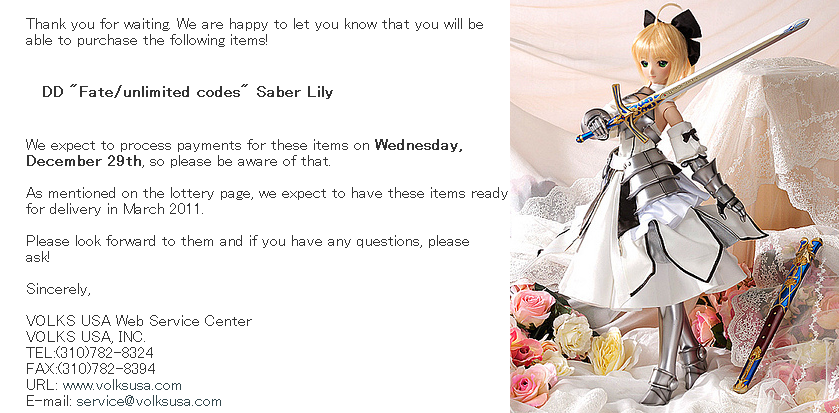The image depicts a promotional sales post from VolksUSA advertising the availability of the "DD Fate Unlimited Codes Saber Lily" doll. On the right side of the image, there's a detailed photograph of the doll, styled as a warrior princess. She has long blonde hair with bangs, piercing dark eyes, and a large black bow adorning the back of her head. She is dressed in an intricately designed white satiny dress featuring a body armor corset, silver boots, and holding a long silver and blue sword. She wears silver pantyhose and high heels, and the setup includes pink, white, and yellow roses at her feet alongside white silky fabric and soft pink and white lace curtains in the background.

The text on the left side of the image reads: "Thank you for waiting. We are happy to let you know that you will be able to purchase the following items: DD Fate Unlimited Codes Saber Lily. We expect to process payments for these items on Wednesday, December 29th, so please be aware of that. As mentioned on the lottery page, we expect to have these items ready for delivery in March 2011. Please look forward to them. If you have any questions, please ask. Sincerely, VolksUSA Web Service Center, VolksUSA, Inc., Telephone 310-782-8324, Fax 310-782-8394, URL www.volksusa.com, email service@volksusa.com."